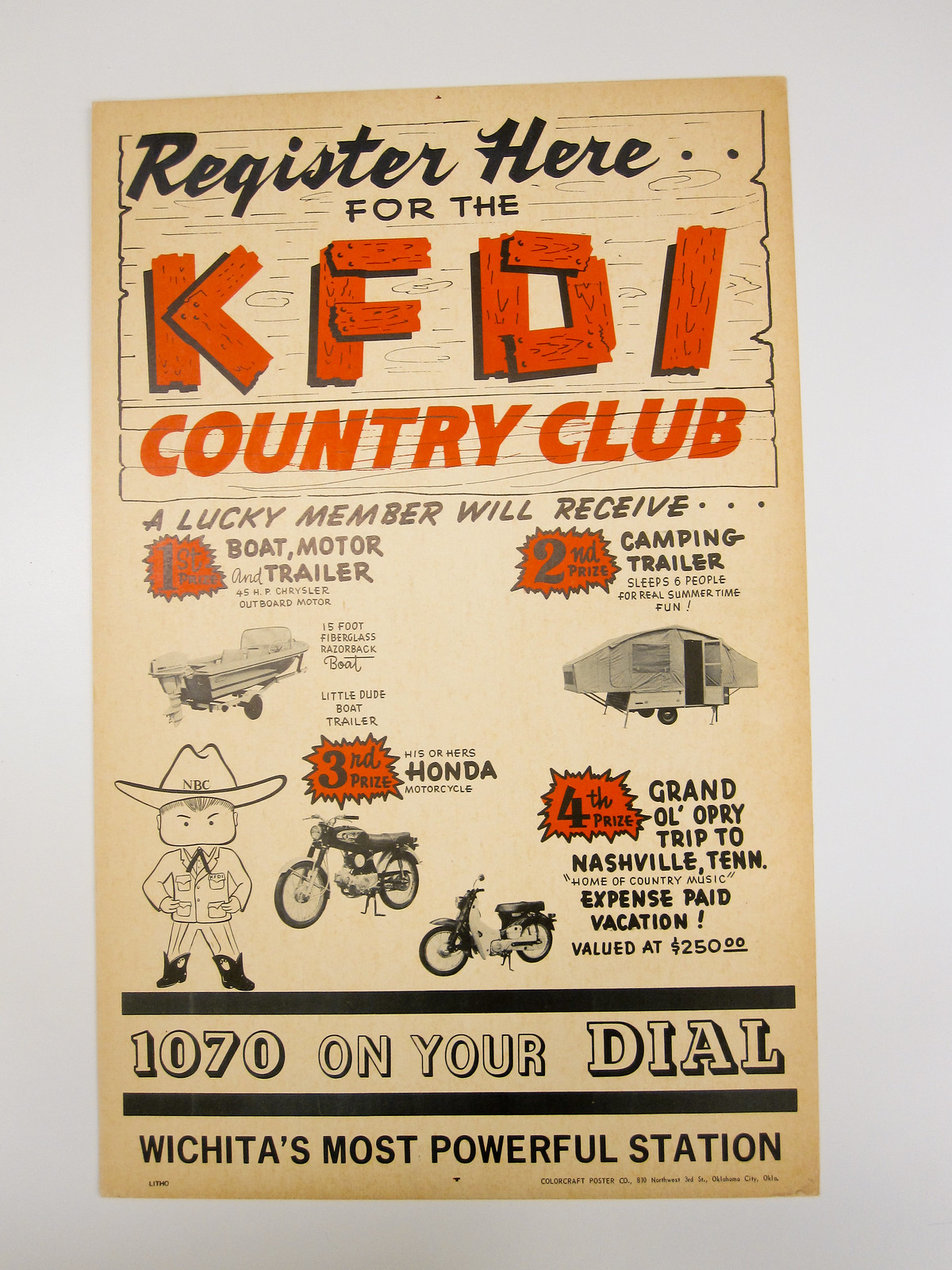This vintage poster, printed in black-and-white with spot color, is affixed to a gray wall background and dates back to the 60s or 70s. It serves as an advertisement for the KFDI Country Club registration. The top of the poster features the text "Register Here" in black script, followed by the organization's name, "KFDI Country Club," in a striking, orange wood-style font. Just below, in light gray type, it reads "A Lucky Member Will Receive..." with an array of four prizes listed in orange conversation bursts with black text: 

1. First prize: a boating motor trailer, depicted with a black-and-white photo.
2. Second prize: a camping trailer, also shown in a black-and-white photo.
3. Third prize: a Honda motorcycle, illustrated with a photo of two scooters. 
4. Fourth prize: an all-expenses-paid trip to the Grand Ole Opry in Nashville, Tennessee, valued at $250.

Adjacent to these prize descriptions is a cartoon drawing of a sheriff in a western outfit with hands on hips, standing next to the motorcycle illustration. At the bottom of the poster, the text confirms the affiliation with KFDI 1070, Wichita’s most powerful radio station, with the phrasing "1070 on your dial." The overall style exudes a nostalgic print publication aesthetic.